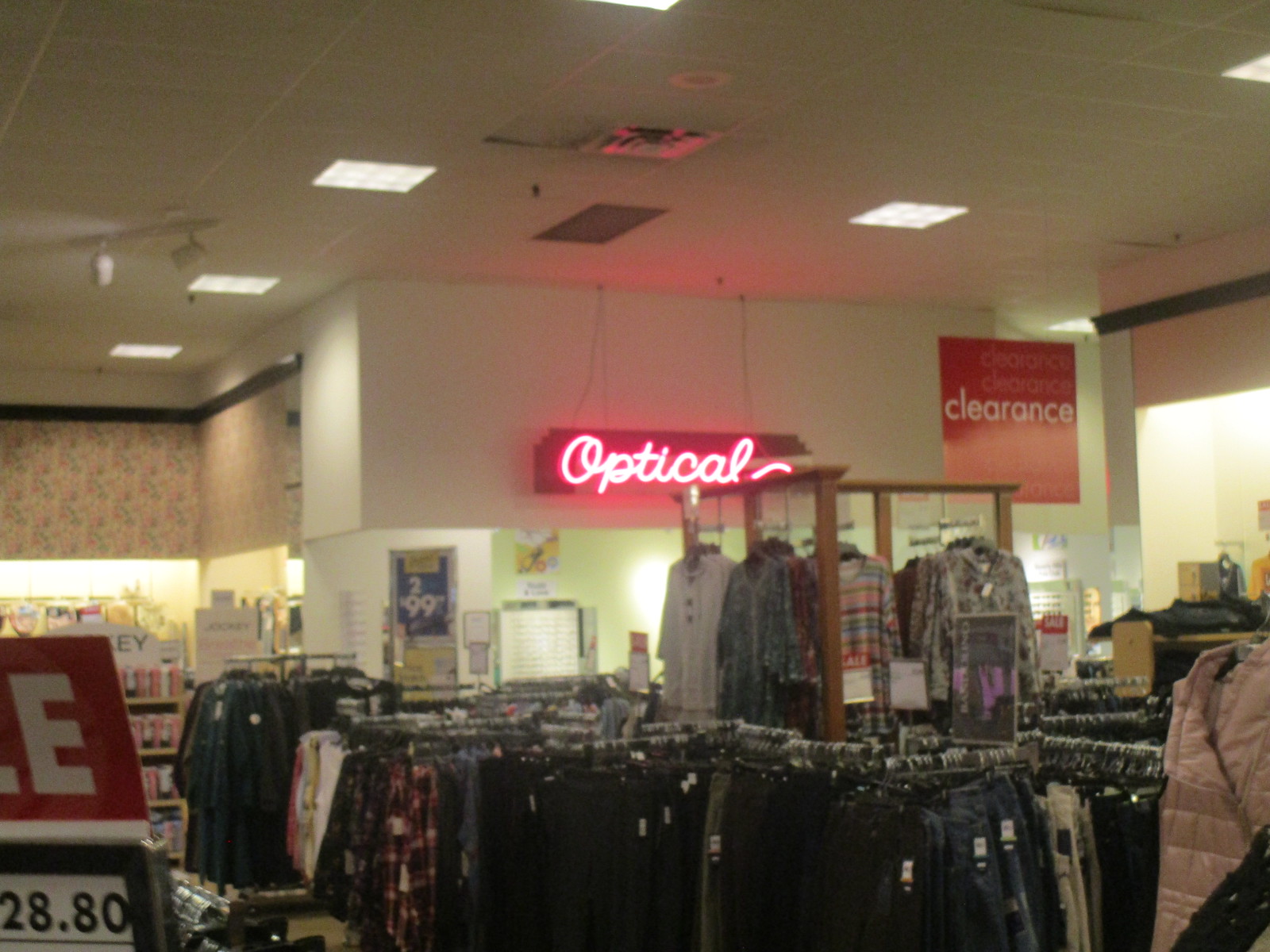A faded, vintage-style photograph of a busy department store, evocative of a TJ Maxx or Ross, captures a clothing section dominated by a prominently highlighted "Optical" area. The sign above the optical section reads "2 for 99," suggesting a glasses discount, though the details are somewhat obscured by the aged quality of the image. Below the sign, a small rack seemingly holds glasses, perched next to a noticeable clearance sign. The store is filled with hanging clothing, predominantly shirts displayed at a higher level, with various pants scattered around. From the left side of the photograph, a sale sign protrudes, adding to the bustling retail atmosphere.